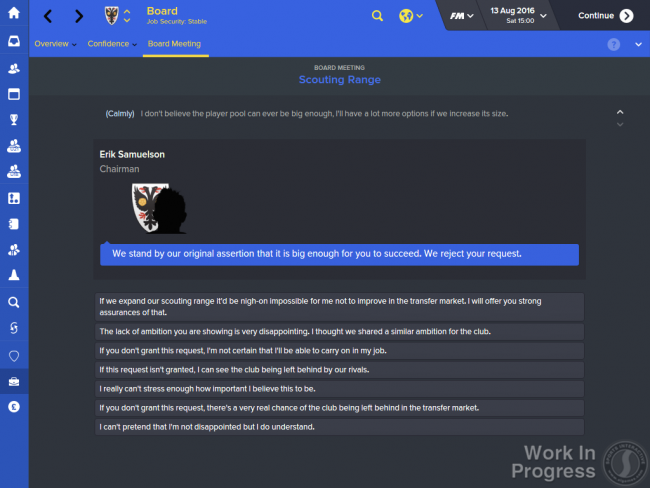In this detailed image from a soccer management simulation game, the interface prominently displays a critical in-game decision. At the top of the screen, the game board indicates the player's job security status as "Stable," with the in-game date and time set to Saturday, August 13, 2016, at 15:00 (3 PM). 

The main section is focused on "Scouting Range," suggesting a strategic discussion about expanding the club's ability to scout new talent. The player's dialogue reads: "I don't believe the player pool can ever be big enough. I'll have a lot more options if we increase its size." In response, Eric Samuelson, identified as the chairman, states: "We stand by our original assertion that it is big enough for you to succeed. We reject your request."

Following this exchange, the player is presented with several response options:
1. Expand our scouting range. It would be nigh on impossible for me not to improve in the transfer market. I will offer you strong assurance of that.
2. The lack of ambition you are showing is very disappointing. I thought we shared similar ambition for the club.
3. If you don't grant this request, I'm not certain I'll be able to carry on in my job.
4. If this request isn't granted, I can see the club being left behind by our rivals.
5. I really can't stress enough how important I believe this is.
6. If you don't grant this request, there is a very real chance of the club being left behind in the transfer market.
7. I can't pretend that I'm not disappointed, but I do understand.

On the left side of the screen, a vertical menu bar provides navigation to various sections such as Overview, Confidence, Board Meeting, among others. 

In the bottom right corner, a watermark indicates that this version of the game is still in development, marking it as a beta version and not the final release. This image captures a nuanced moment where the player must navigate boardroom politics to expand scouting capabilities while testing an unreleased version of the game.